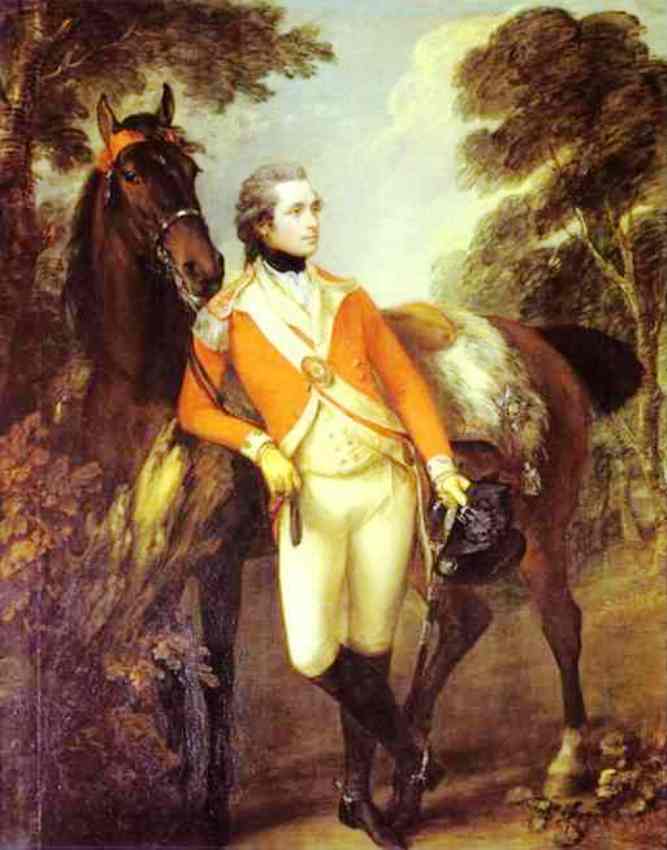This painting portrays a distinguished man standing in front of his horse, exuding a composed yet commanding presence. The central figure, with neatly tied, braided gray hair, gazes forward and slightly to the right. He wears an elaborate military uniform featuring a golden or possibly bright orange vest adorned with intricate buttons, a black collar, a white shirt, white pants, and knee-high black boots. A red bandana adorns his neck, contrasting with his somewhat pale complexion. In his left hand, he holds what appears to be a dark-colored hat or helmet.

The man leans gently on his right elbow against the head of his noble horse, which stands slightly behind him. The horse, a dark brown steed with a big black tail, has its head turned to face forward and right, looking over the man's shoulder. The horse's attire includes a notable beige blanket or fur saddle and a cloth piece that stretches between its ears. The scene is enveloped in a serene landscape; bushes and possibly flowers of purple and yellow hues grow from the bottom of the painting in front of the horse's left hoof. Rocks dot the brownish dirt ground they stand upon. 

In the background, the painting captures a blue sky with wispy clouds, framed by trees on both the left and right sides of the canvas. The pastoral and timeless feel suggests a setting reminiscent of the Renaissance or Middle Ages, encapsulating a moment of restful contemplation for the horse and rider, both seemingly engrossed in the same distant view.